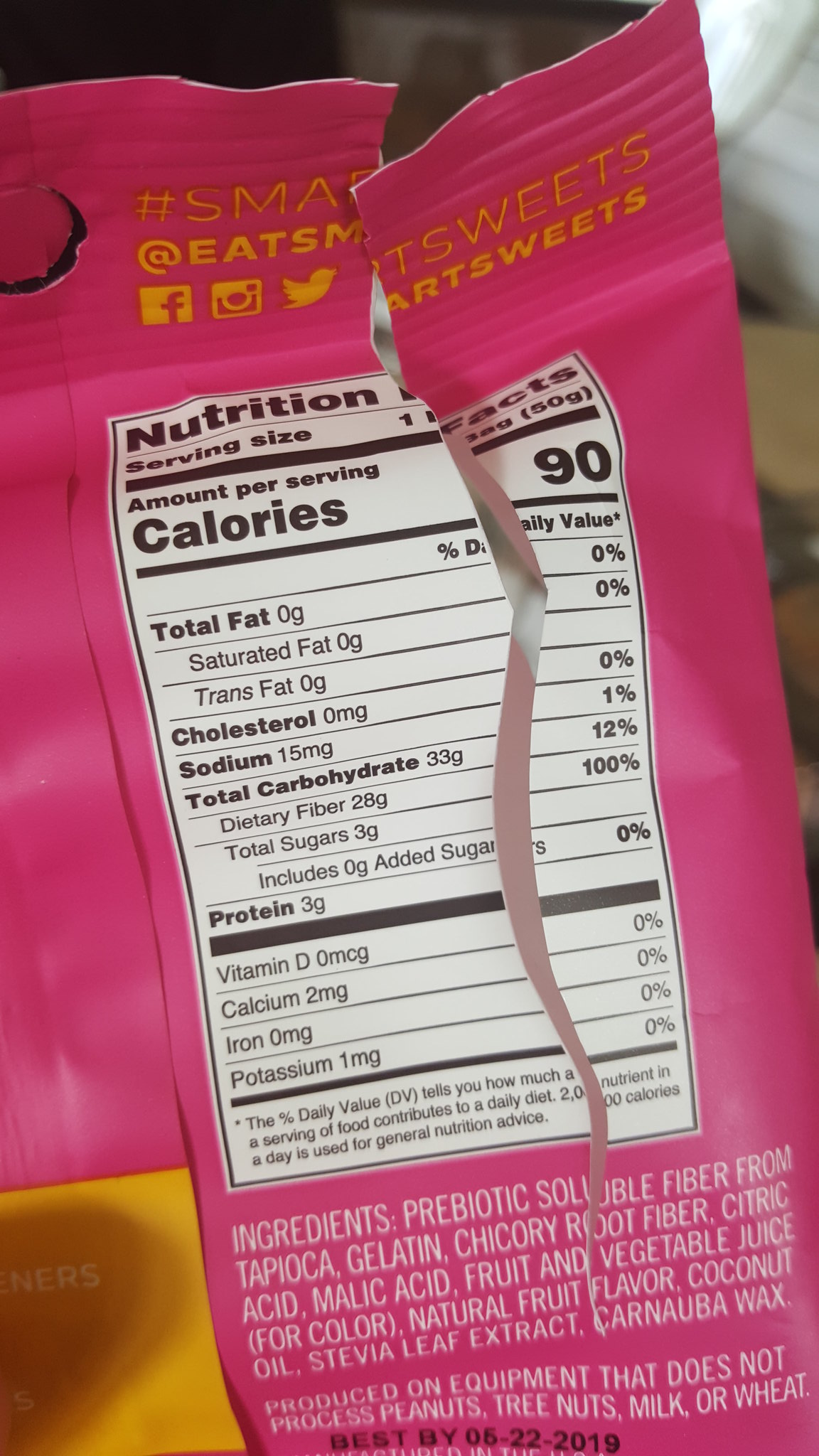The image depicts the back of a bright fuchsia-colored bag of Smart Sweets that has been torn open down the middle, likely after all the sweets inside were consumed. The bag is photographed in a typical household setting, with blurred background details suggesting it was taken on a phone. The torn edge reveals the detailed nutrition label and ingredients list. The orange text at the top of the bag reads "Eat Smart Sweets," accompanied by social media icons of Facebook, Instagram, and Twitter with the handle @eatsmartsweets. The nutrition facts indicate each serving contains 90 calories, 0 grams of total fat, 0 milligrams of cholesterol, 15 milligrams of sodium, 33 grams of total carbohydrates (including 28 grams of dietary fiber and 3 grams of total sugars with 0 grams of added sugars), and 3 grams of protein. It also notes that the bag provides 0% of daily Vitamin D, 2 milligrams of calcium, 0% of daily iron, and 1 milligram of potassium. The ingredients list and the "Best By" date, denoted as 06-22-2019, are located at the bottom of the label.